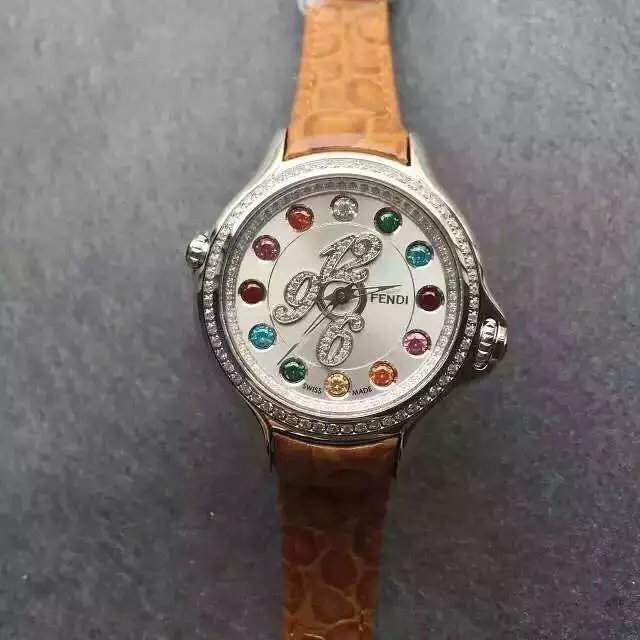A professionally staged photograph showcases an intriguing watch against a grey backdrop, capturing a meticulous attention to detail. The watch is propped up, highlighting its sophisticated aesthetic. The silvery face of the timepiece is adorned with a delicate rhinestone pattern encircling it, while two sleek, silver dials enhance its elegance. The watch's straps, slightly out of focus, exhibit a leathery texture adorned with a subtle, spotted pattern. Where numerical indicators typically reside, various gemstones in shades of purple, dark green, teal, turquoise, and orange replace the numbers, adding a splash of vibrant color. The numerals 12, 9, and 6 are distinctly represented in silver. The time on the watch reads approximately 2:37, completing this detailed and captivating representation of the timepiece.